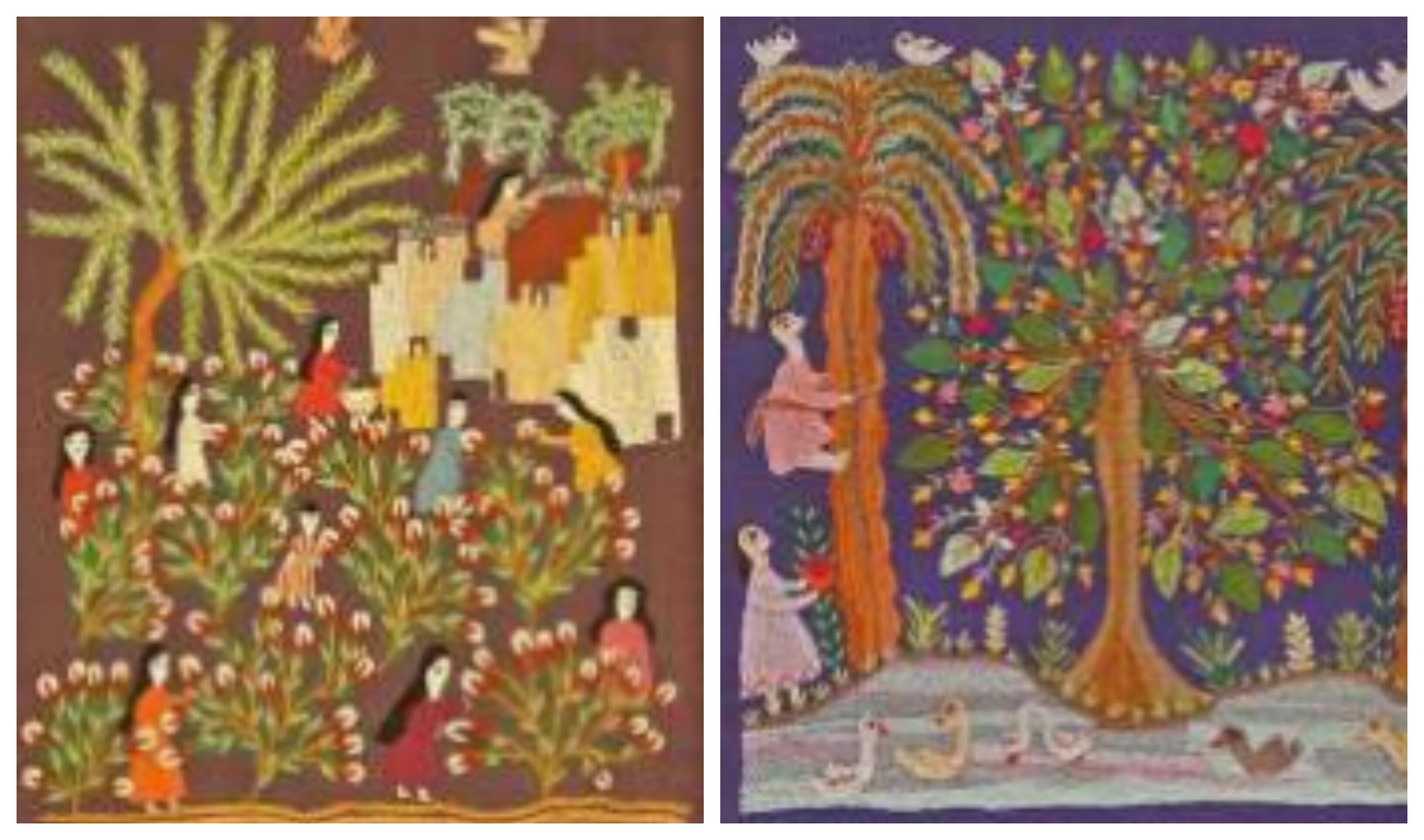The image showcases two faded, hand-woven or sewn artworks side-by-side, resembling old, colorful paintings on fabric. 

The left piece depicts a pastoral scene. A group of women, dressed in vivid colors such as orange, red, pink, yellow, and blue, is harvesting what appear to be lush green plants with white flowers, possibly cotton. In the background, there's an old building, reminiscent of a stone castle, painted in shades of yellow, white, blue, and red. The background colors in this section are predominantly green, white, red, black, orange, yellow, brown, blue, and beige, indicating a rich and diverse color palette.

The right piece features a vibrant, nature-inspired design set against a purple backdrop. This scene includes two tall trees, one resembling a palm or coconut tree with a character in a pink outfit climbing it, and another tree with expansive, vividly colored branches in green, red, yellow, white, and orange. Below, a woman in a pink dress appears to be holding an apple, and there are five birds or geese at the bottom, along with more birds perched atop the trees. The tree leaves form a circular mosaic of colors, adding to the overall dynamism of the scene.

Both images, although minimalistic and lacking facial features, present a tapestry of rural life intertwined with nature, painted with an extensive and lively color scheme.